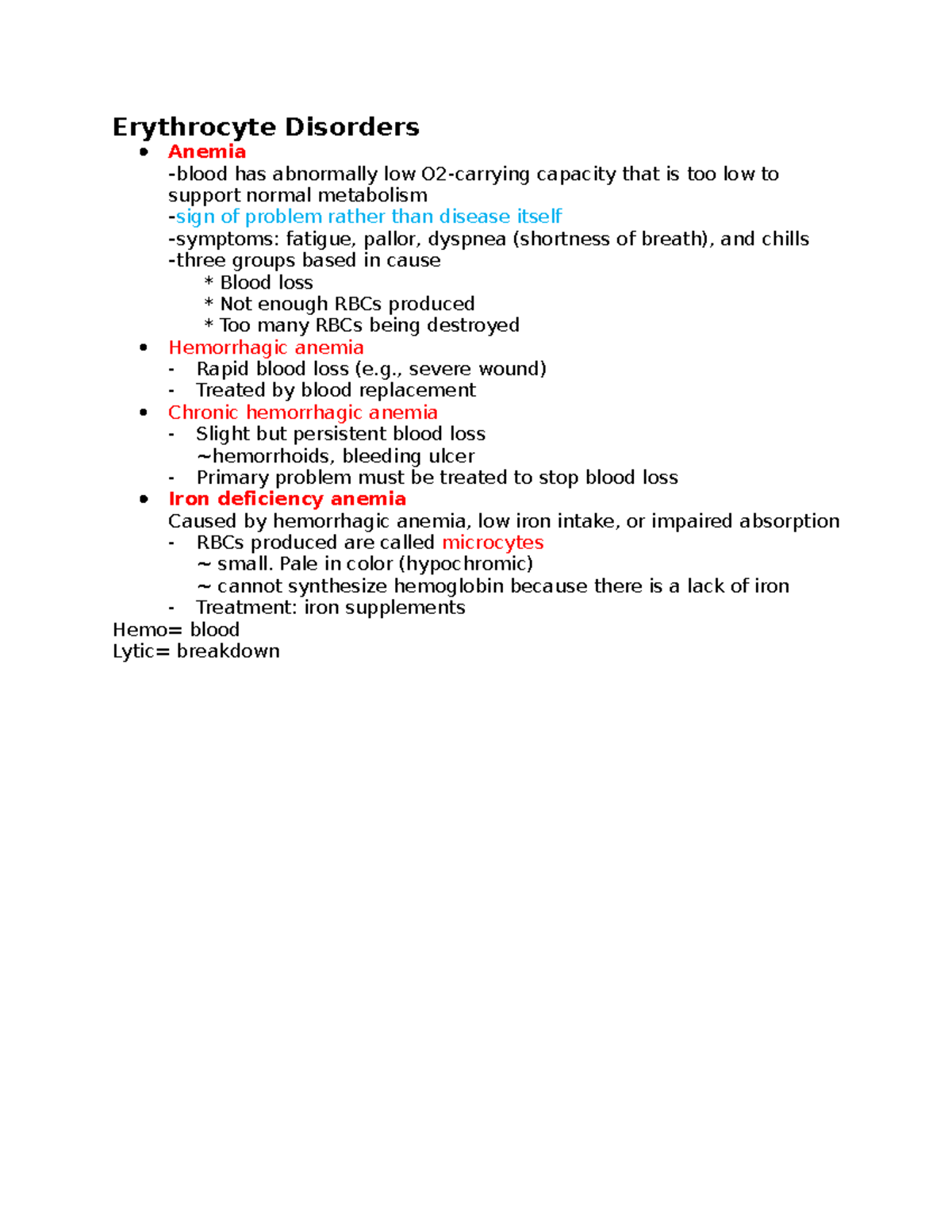**Image Description:**

The image features a white background with various sections of text in different colors and fonts, designed to explain disorders related to erythrocytes. 

At the top, in large, bold black text, the title reads "Erythrocyte Disorders". Below this title, there are four sections with titles in red text, each representing a different type of anemia:
1. Anemia
2. Hemorrhagic Anemia
3. Chronic Hemorrhagic Anemia
4. Iron Deficiency Anemia

Under the title for "Anemia", there is a detailed description that intersperses black and light blue text. The description reads:

- In black text: "Blood has abnormally low O2 carrying capacity that is too low to support normal metabolism."
- In blue text: "a sign of a problem rather than a disease itself."
- In black text: "Symptoms: fatigue, pallor, dyspnea (shortness of breath), and chills."
- In black text: "Three groups based on cause: blood loss, not enough RBCs produced, too many RBCs being destroyed."

Each of the other red-titled sections similarly explains the related conditions, with the use of different textual colors and details.

At the very bottom of the image, in black text, a glossary-like explanation is provided:
- "Hemo = blood"
- "Lytic = breakdown"

The combination of colors and fonts creates a structured and informative chart, making it easier to differentiate and understand the various types of erythrocyte disorders.